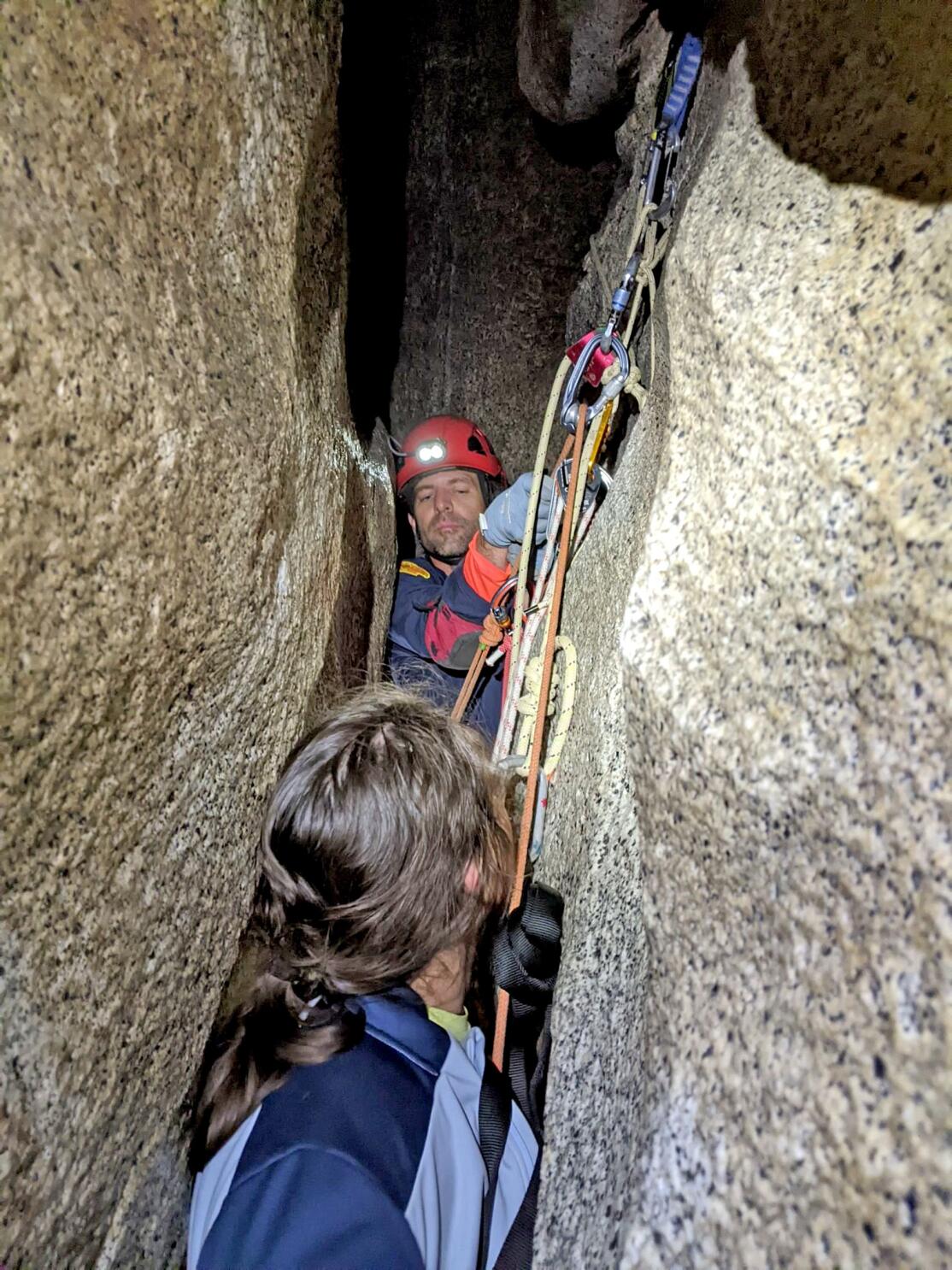This photograph depicts a man and a woman navigating a treacherously narrow passage between two large slabs of rock. The setting suggests either a mountainous area or a cave, with light grayish beige rock walls closely confining the climbers. The man, identifiable by his light skin, wears a red helmet equipped with a headlamp, a blue jacket over an orange shirt, and light blue gloves. He appears to be assisting the woman or engaged in a similar activity, possibly climbing or rescue work. The woman, with long, dark brown hair tied back, is dressed in a light blue and dark blue jacket. Both are tightly wedged between the rocks, emphasizing the narrowness and potential danger of the passage. They are equipped with harnesses of blue, yellow, and orange colors, and various ropes and carabiners are visible, signifying their preparedness for the challenging climb.